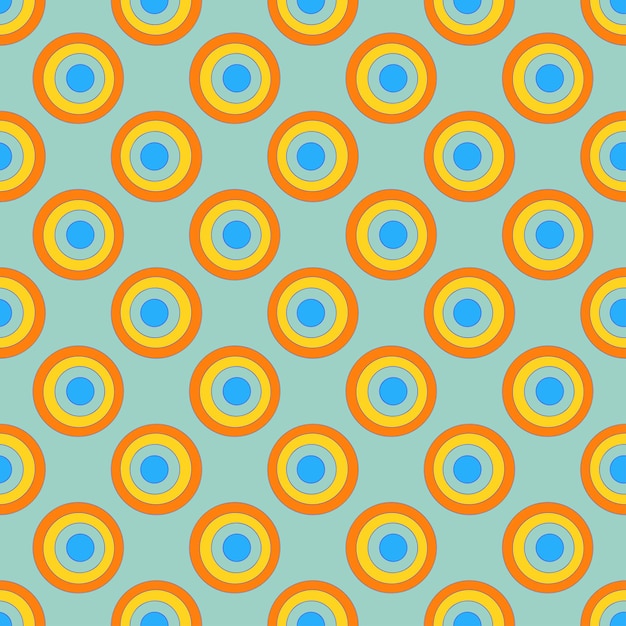The image features a rectangular horizontal layout with a light blue background, covered entirely in a uniform pattern of concentric circles. Each circle consists of four distinct color bands: an outermost border of orange, followed by a yellow ring, a light blue ring, and a central dark blue circle. The circles are identical and arranged in rows that offset slightly with each other, creating diagonal alignments across the image. The edges of the picture cut off portions of certain circles. This consistent, repetitive design could resemble patterned wallpaper.